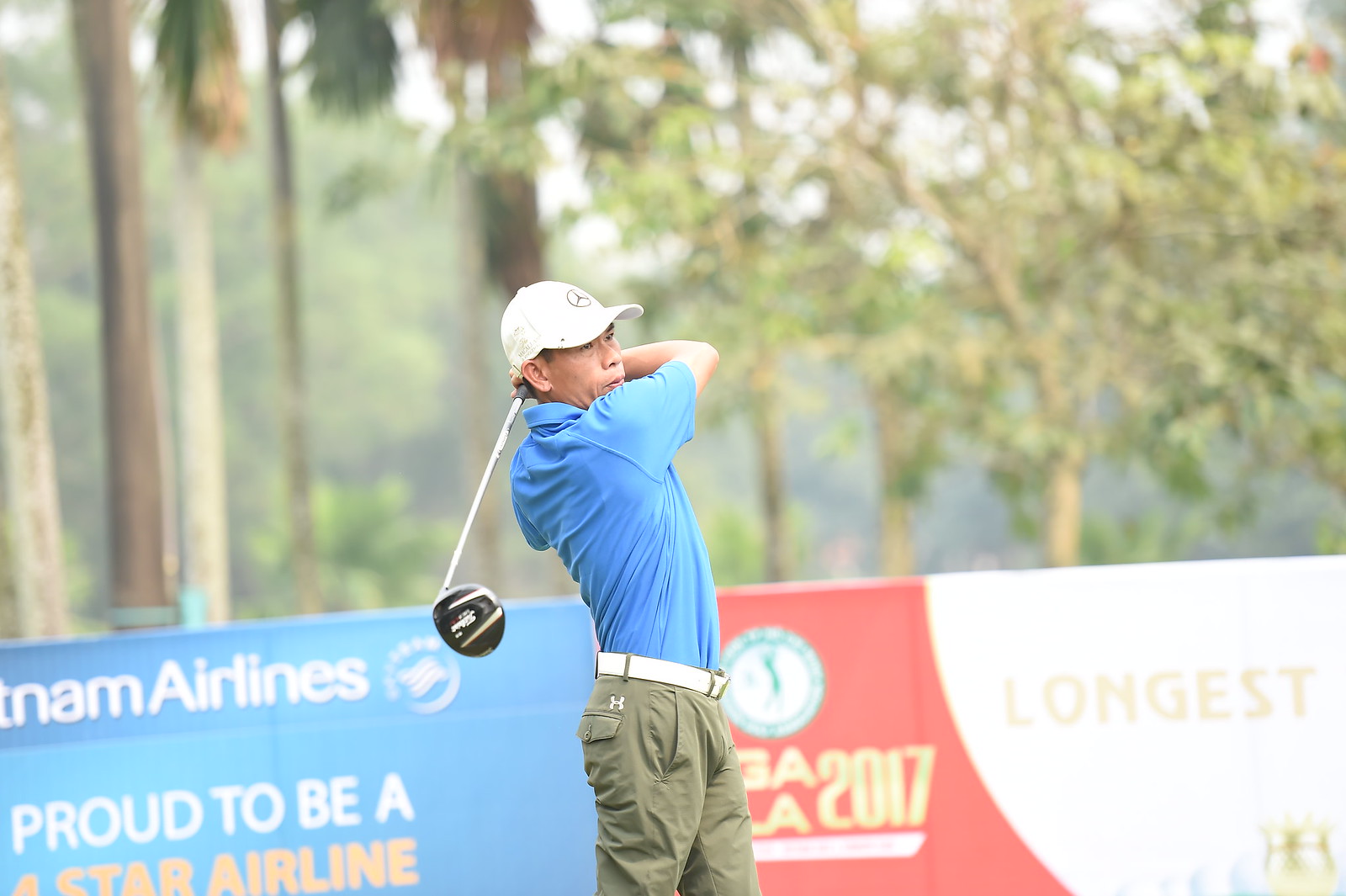The image captures a vibrant scene from a daytime golf tournament. Dominating the foreground is a player mid-swing, wearing a blue polo shirt tucked into green khakis secured with a white belt. His white baseball cap, adorned with the Mercedes logo, shades his face as he executes a powerful shot, his golf club—a silver shaft with a large, black head—arcing behind him. The man’s attire and focused posture suggest a professional or serious amateur golfer. In the background, the setting is lush with numerous trees under a clear sky, enhancing the outdoor sports atmosphere. Various sponsor banners are visible, including one prominently displaying "Vietnam Airlines, proud to be star airline," and another with partially legible text mentioning “GALA 2017” and “Longest.” These indicators collectively hint at a well-organized and possibly high-stakes event.